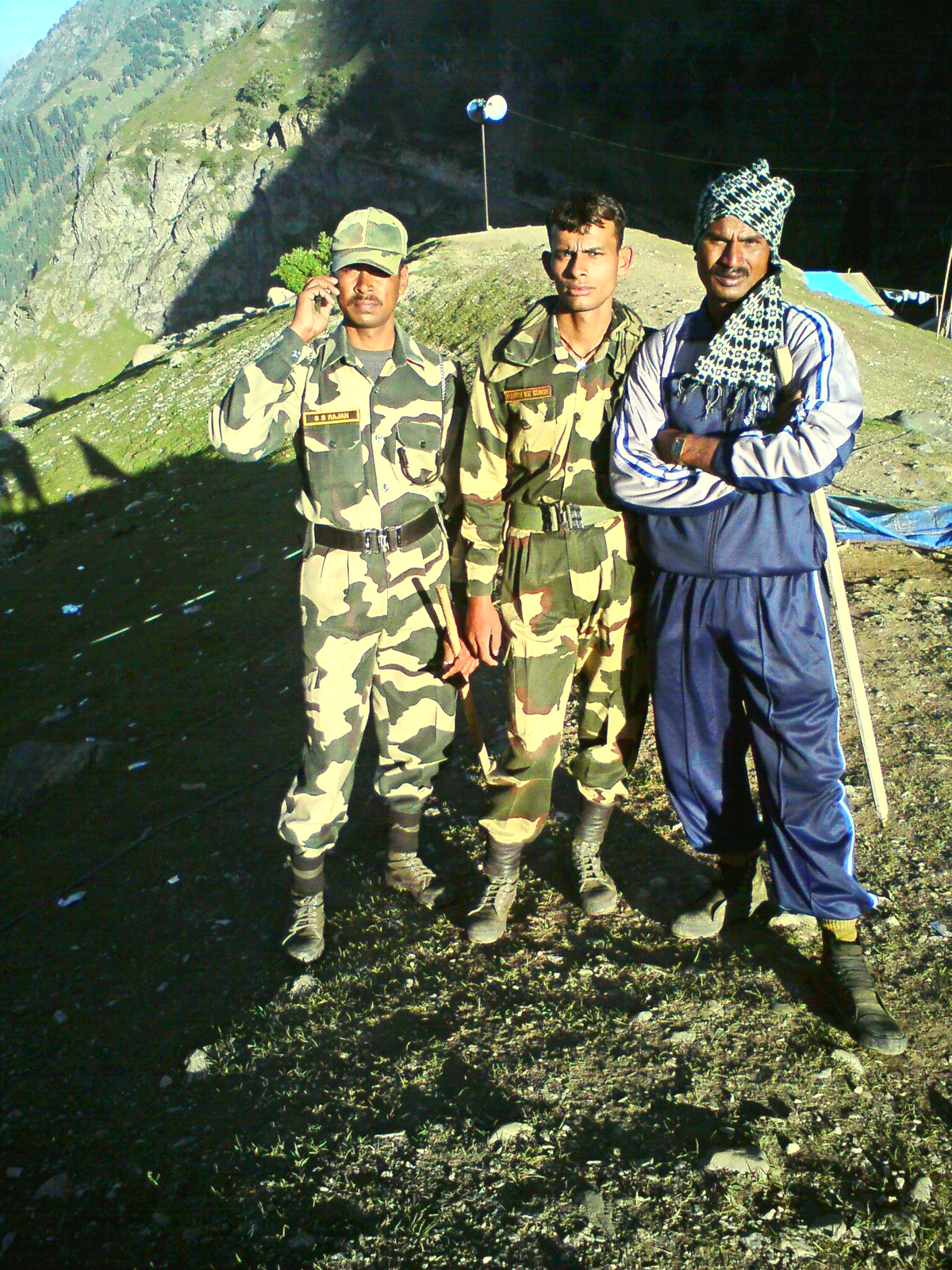This vertically aligned rectangular image, devoid of a border, captures a detailed scene featuring three men posing on a rugged mountain top. In the background, there are steep mountain inclines under a sliver of blue sky visible in the upper left corner, while a pole with an attached light stands out.

The man on the left is in a darker camouflage uniform complemented by a ball cap of the same pattern, a brown mustache, and darker skin. Beside him, the middle man also wears a camouflage uniform—this one lighter in color—with no hat, revealing his short black hair and similarly darker skin. Both men have name tags, though they are illegible.

The third individual on the right contrasts sharply with his companions, dressed in blue pants and a blue and gray long-sleeve tracksuit top, adorned with stripes along the arms. He also sports a scarf wrapped around his head, has darker skin, and a black mustache. His stance, with arms crossed and a walking stick in his left hand, suggests a native connection, perhaps indicating the setting is Afghanistan.

The picture, taken during daylight, nonetheless features dark shadows that obscure parts of the background, creating a dramatic contrast with the bright sunlit area visible in the upper left corner. The trio stands on rocky terrain with a small hill behind them, capturing the rugged, perhaps desert-like, military environment.